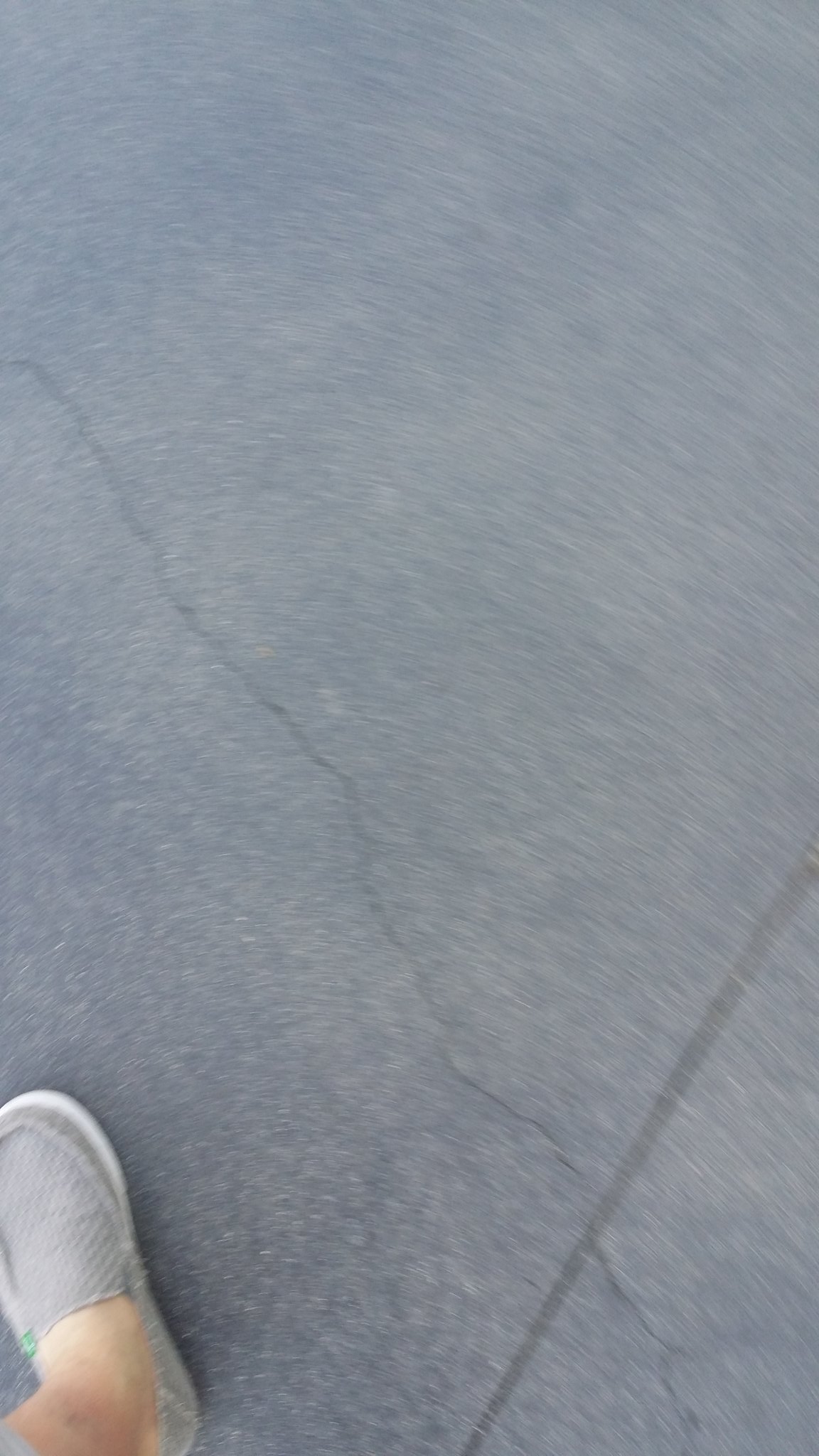The image shows a stretch of gray asphalt seen from an overhead perspective. The surface has a relief indentation running across it, intersected by a prominent crack. The lighting suggests it is daytime, though the overcast sky casts the scene in muted, gray tones without any bright illumination. In the lower left-hand corner of the image, a foot is visible, clad in a gray moccasin featuring a white insole. The moccasin covers a somewhat thick ankle, and the person is wearing bluish-gray capri pants, revealing a portion of their shin. The overall composition is minimal, focusing primarily on the textured asphalt and the lone foot.